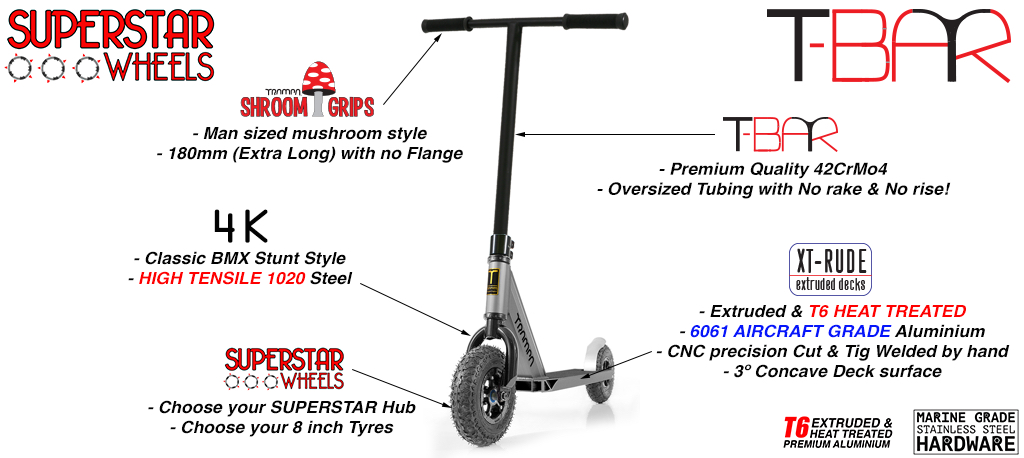The advertisement features a gray electronic-powered scooter bike prominently displayed against a white backdrop. The scooter boasts black handlebars and a footrest, complemented by black wheels. At the top left of the ad, the text "Superstar Wheels" is highlighted in red, while the top right features "T-Bar" in black and red text. Arrows and labels meticulously point to various parts of the scooter, providing detailed descriptions of its features. The handlebars are equipped with “Shroom Grips,” described as man-sized, mushroom-style grips that are 180mm extra long and flangeless, illustrated with a red and white mushroom icon. The oversized T-Bar, made from premium quality 42CRMO4 tubing, is noted for having no rake and no rise. Near the wheel, which is part of the scooter’s BMX stunt-style feature crafted from high-tensile 1020 steel, the ad invites users to "choose your superstar hub" and "choose your 8-inch tires." Additional text at the bottom right of the ad includes logos, one indicating "Marine Grade Hardware." Another logo features the letters "TG" with some accompanying, yet hard-to-read, text, further emphasizing the quality components from various brands used in the scooter's construction.